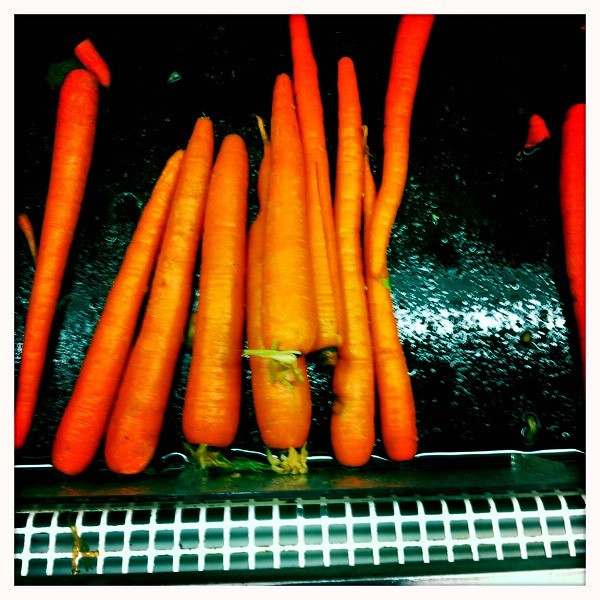The image features a shiny, black, and possibly metallic surface with water splashes on it, creating a wet or greasy appearance. Below this surface, extending almost the entire length of the bottom of the picture, is a white grate composed of small square patterns, seemingly made of hard plastic. 

On top of the black surface, there is a cluster of approximately nine to eleven large and somewhat reddish-orange carrots. These carrots are arranged mostly in an up-and-down orientation, with some overlapping each other. A few of the carrots retain their green leaves at the tops, while others show black discoloration. They appear unwashed and unpeeled. 

Notably, a single carrot lies isolated on the far left, with its tip broken off and positioned near its top. Another carrot on the far right is only partially visible, cut off at the edge of the frame. In the middle, there is a noticeable gap where the black surface is visible without any carrots.